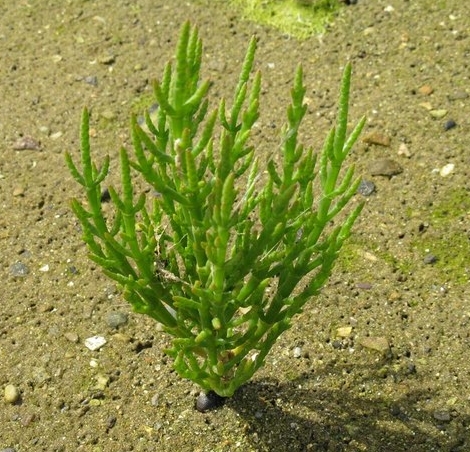The image depicts an outdoor scene with a rugged, rocky surface that has a mix of greenish and brownish hues. Scattered throughout the soil are various pebbles and larger rocks, including a brown one, a black one, a rust-colored one, and a smaller white rock. At the center of the picture, a distinctive aquatic plant is growing, reaching upwards with lime-green stalks that resemble spears. Each spear forks off into smaller branches that diagonally angle left and right, ending in rigid tips. This plant, reminiscent of underwater flora, casts a shadow to the right, indicating the light source is coming from the top left corner. Around the main plant, patches of green moss can be seen, adding to the texture and color diversity of the rocky surface.